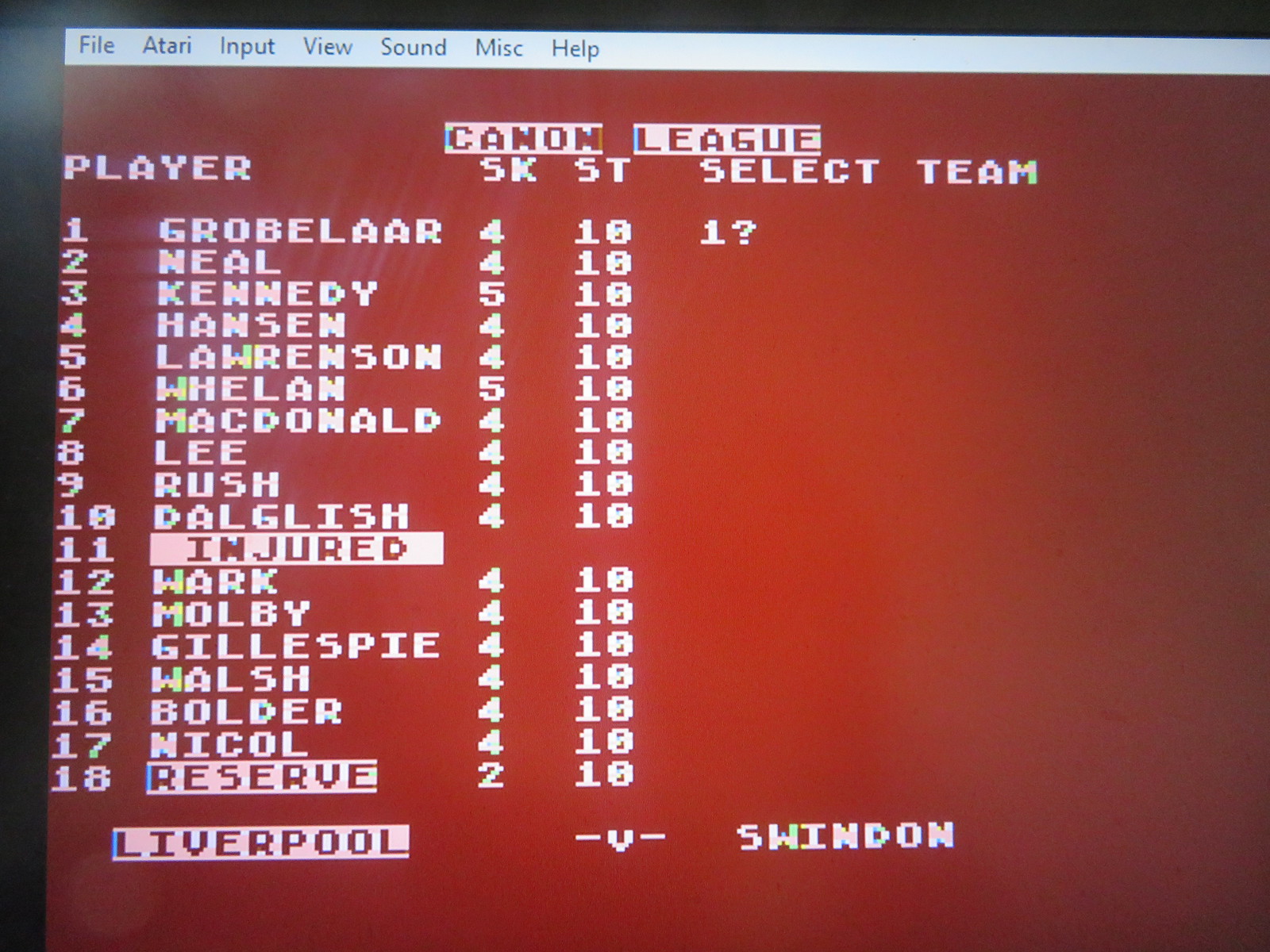The image features a screenshot of an Atari video game, likely soccer-related, displayed on a computer screen. The background is predominantly maroon red with a very light blue strip on top and some black detailing on the top and left sides. The top menu bar includes options such as File, Atari, Input, View, Sound, Miscellaneous, and Help, written in black computer font. Below the menu, there is white text detailing a roster-building screen with 18 player slots, each filled with player names. Notably, slot 11 is marked "injured," and slot 18 is marked "reserve." At the bottom, the team "Liverpool" is highlighted against a subheading for "Swindon." The image's colors include shades of red, black, grey, and off-white, filling the screen entirely without any other objects present. The text "Canon League" and "SKST select team" further indicate that the screen is preparing or managing a sports team.